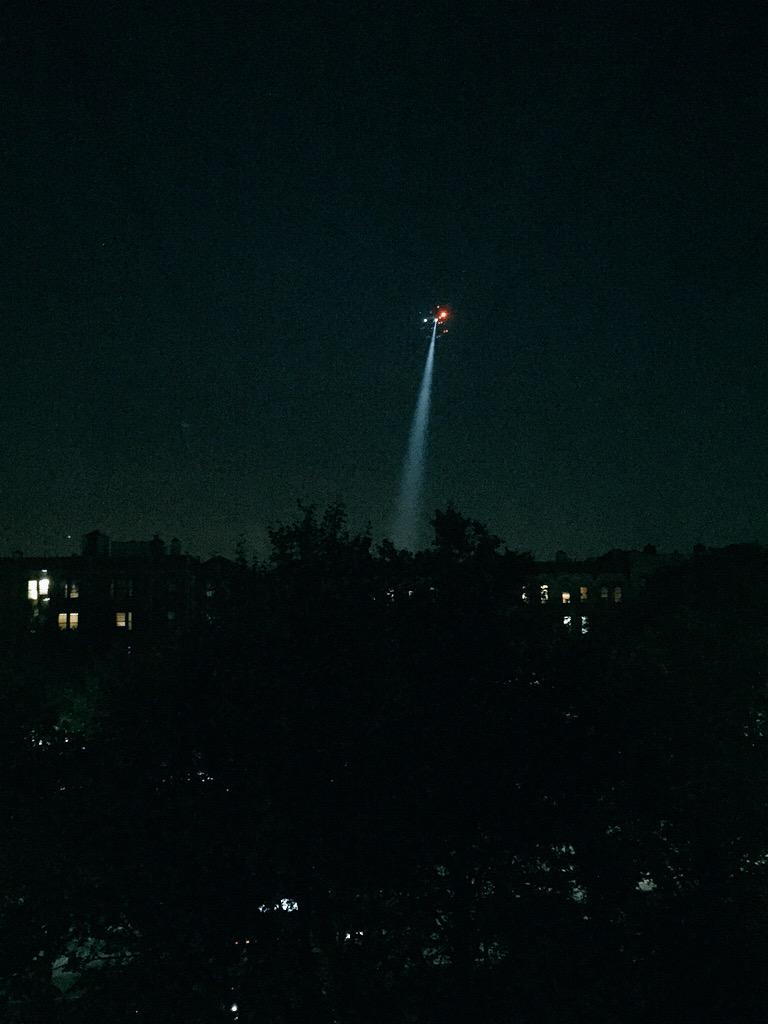The photograph, taken at nighttime, features a helicopter illuminating the scene with a prominent searchlight. The sky is nearly pitch-black, transitioning to a very dark blue near the horizon, likely tinged with some light pollution from a distant city. The bottom half of the image depicts a dimly lit landscape with a few visible houses, their windows glowing softly. The outlines of several trees are discernible, silhouetted against the faint light. Within the sky, the helicopter is equipped with multiple lights on its running boards and front, including a noticeable red light. A powerful beam of light emanates from the helicopter's underside, becoming more diffused and dim as it extends toward the ground. The scene also suggests a reflective surface at the bottom, possibly water, capturing the subtle reflections of the trees above.